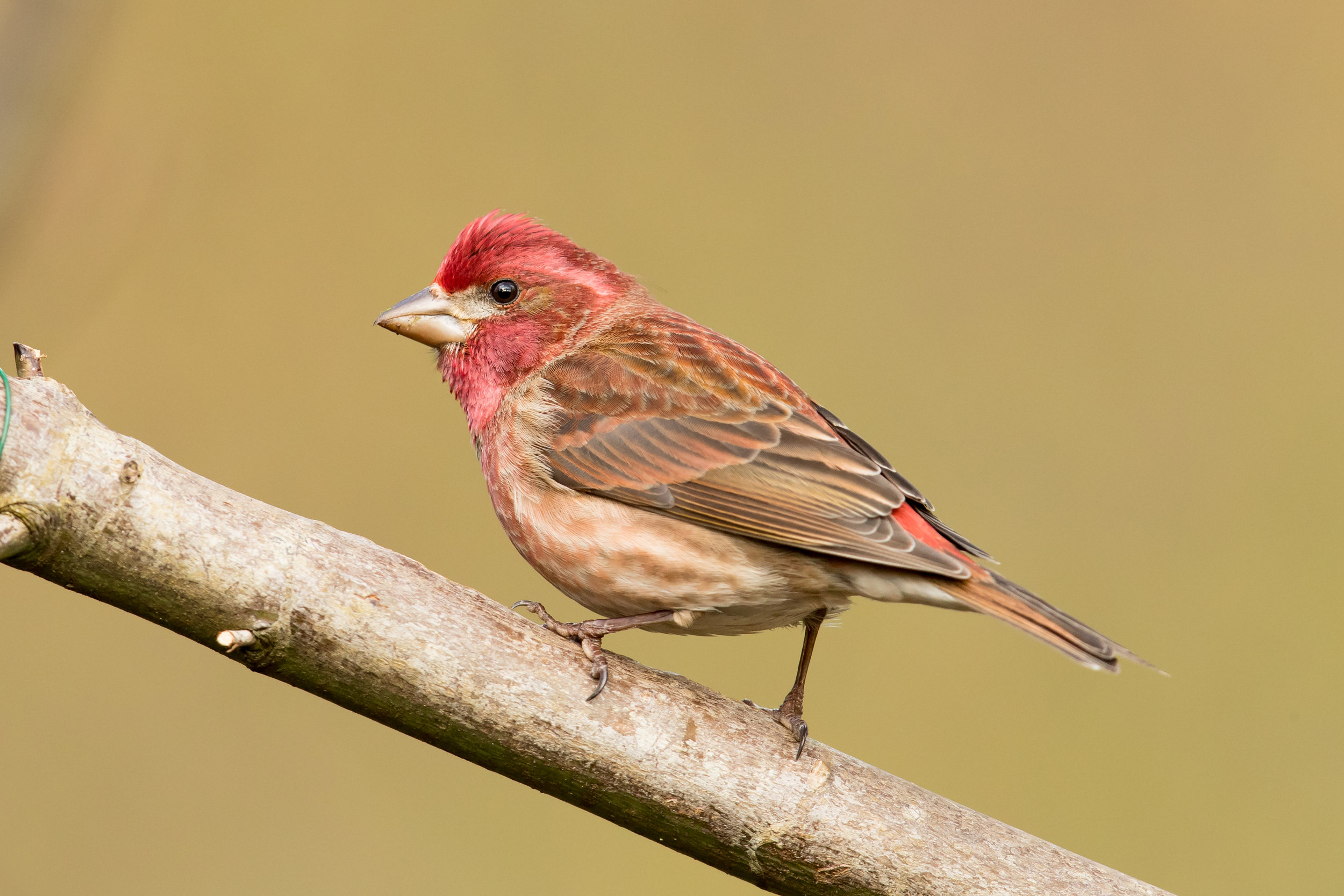This high-definition color photograph, possibly taken by a wildlife photographer, captures a very close-up view of a small bird, likely a finch or a type of sparrow, perched on a single, slightly crooked tree branch. The branch, extending from the lower right to the middle left, features some small, cutoff offshoots and exhibits a wooden, natural hue. The backdrop is a plain, blurred brown, highlighting the bird in sharp focus in the foreground.

The bird itself is diminutive, featuring a vibrant red head with varying shades resembling burgundy, and accented by bright, black beady eyes. It has a light brown beak and dark brown talons standing firmly on the branch. The bird’s wings showcase an intricate pattern of red, brown, and black feathers, while its lower body features white and brown stripes, giving it a somewhat tiger-like appearance. Its tail feathers fan out in a blend of white, red, and black at the end. The bird is facing leftwards, presenting a detailed and striking profile against the unobtrusive brown background.